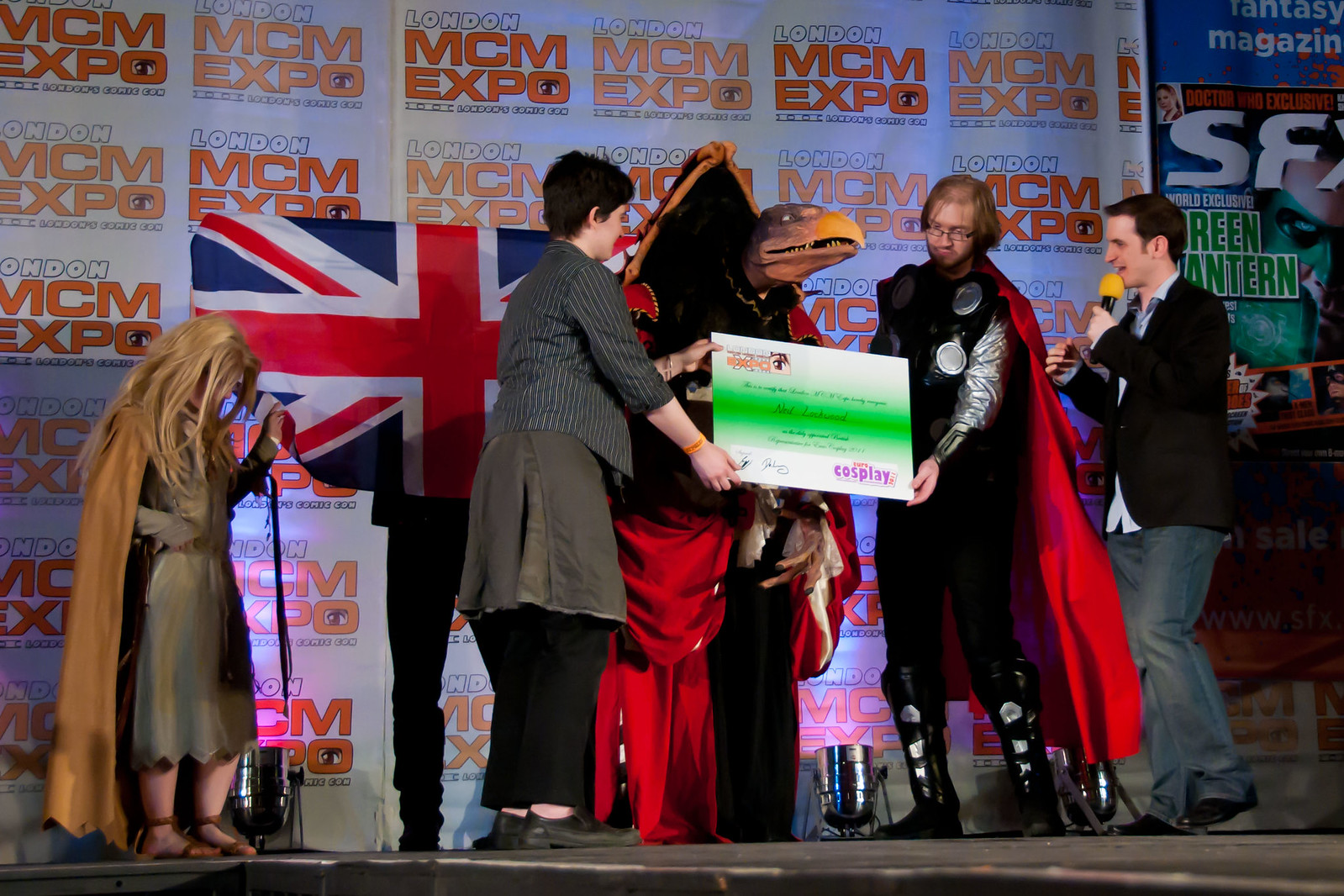The image captures a vibrant scene on stage at the London MCM Expo, where a cosplay presentation is taking place. At the center of the stage, there is a large sign addressed to "Neil Lockwood" that reads "First Cosplay," held by a man in a black and silver medieval-themed costume and a woman in a regular outfit consisting of a long sleeve shirt, skirt, and black pants. Near the center background, a figure in an elaborate vulture costume featuring a red robe stands prominently, possibly referencing a character from the Dark Crystal series. To their right, a man dressed as Thor, identifiable by his long blonde hair and cape, stands holding the British flag—blue with a red and white X and cross. Another man, who is holding a microphone with an orange top, wears a black jacket and blue jeans, seemingly narrating or moderating the event. Furthermore, a small girl dressed in a tan cape, green-gray dress, and brown sandals stands to the far left, looking downwards, adding to the ensemble's diverse character representation. The stage itself features a black hard surface with a silver lining and a gray side, accentuating the colorful and detailed costumes of the participants. The backdrop is adorned with patterns that read "London MCM Expo," reinforcing the event's location, while the British flag held by one of the participants further emphasizes the setting.